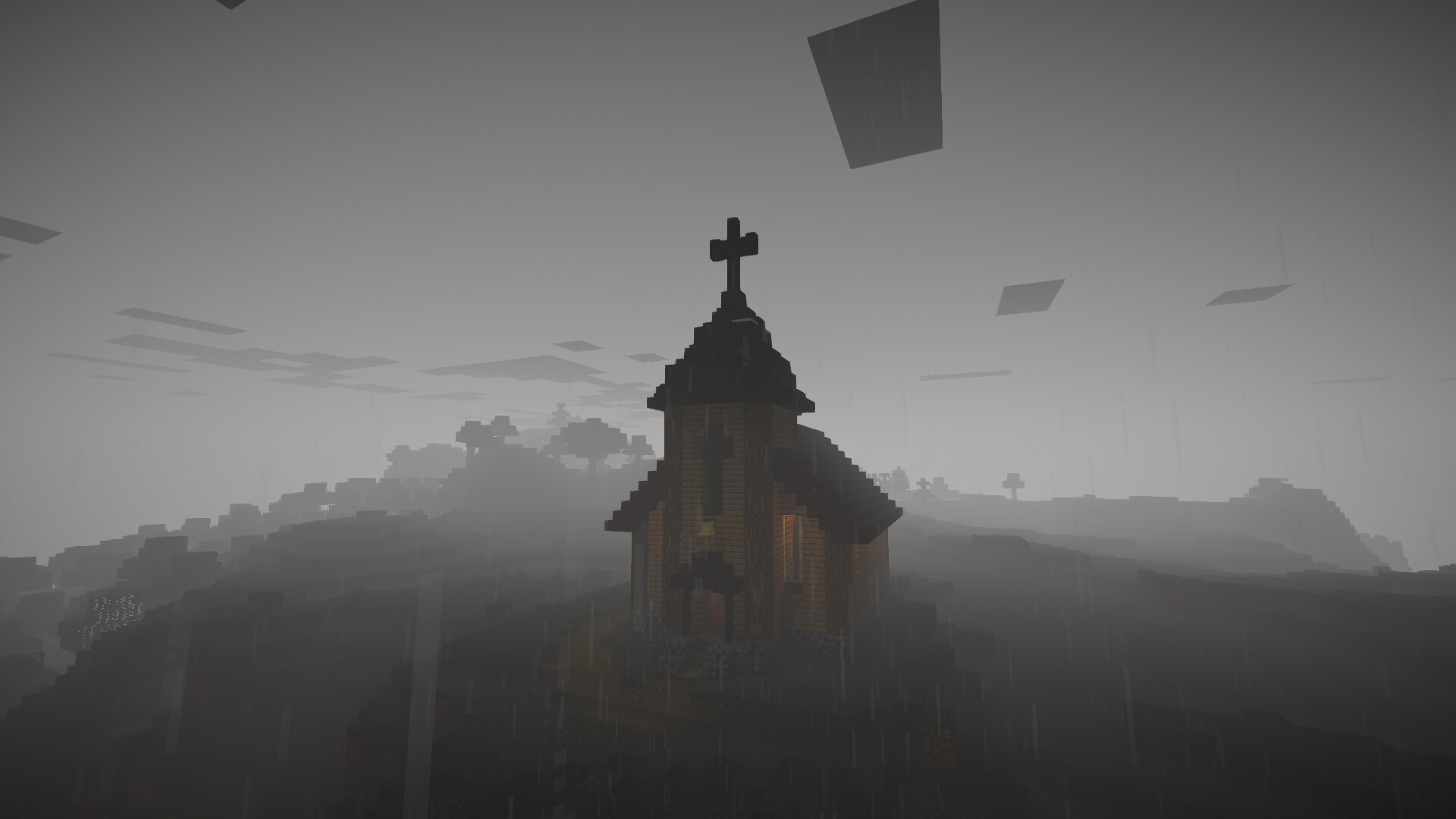At dusk, with a gray, slightly illuminated sky, black rectangular shapes hover ominously. The scene exudes the ambiance of a computer game. It features a wooden church with distinct architectural details. The gable roof, also wooden, is topped with a cross, and another cross design adorns the front facade. The exterior boasts rich wooden textures and the entrance is marked by an arched doorway. This quaint church perches atop a small hill, surrounded by a green landscape. Raindrops cascade from the sky, adding a somber, tranquil touch to the atmosphere.